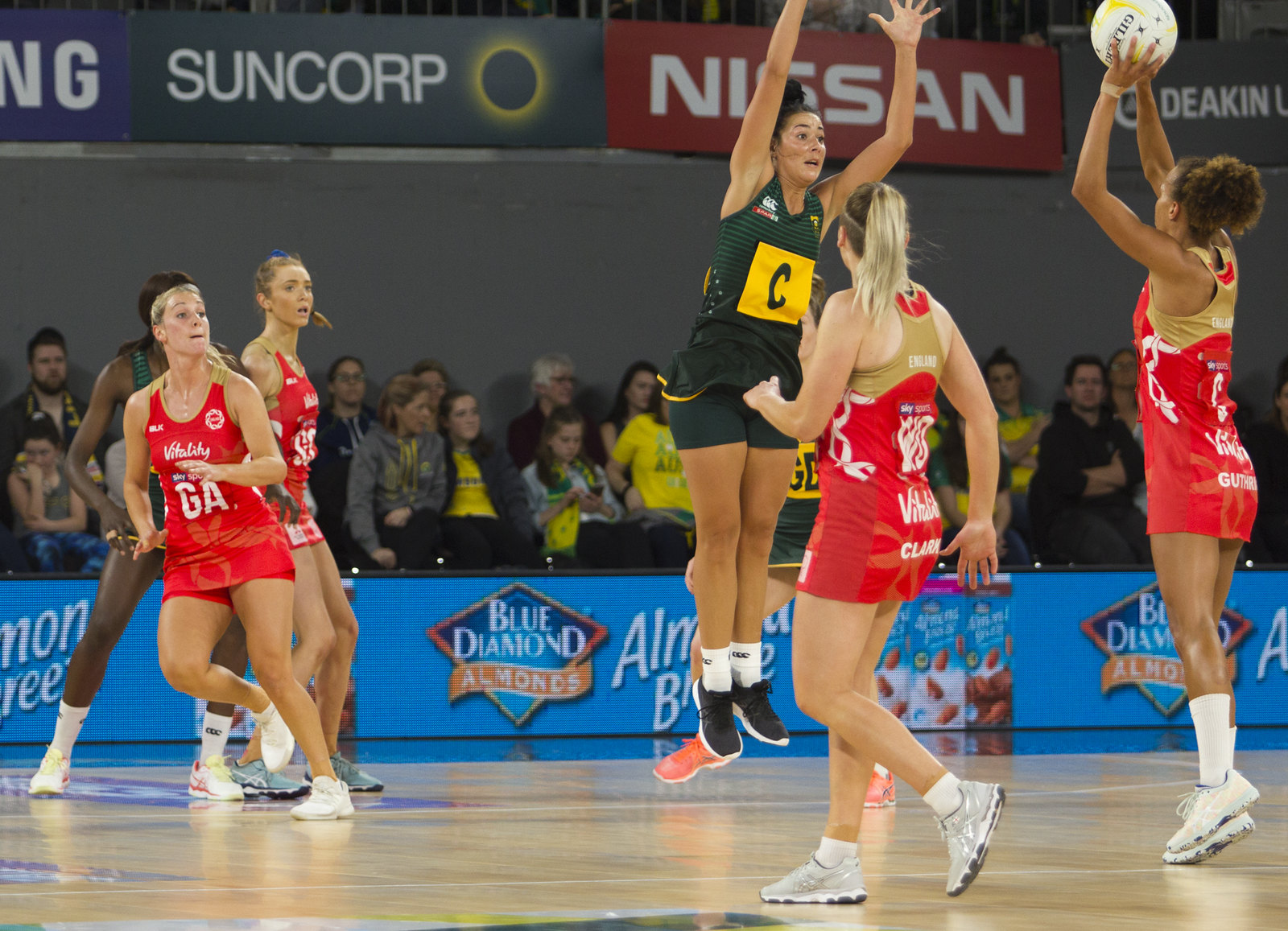This detailed photograph captures the intense action of a women's basketball game played inside a gymnasium auditorium amid enthusiastic spectators. The court is bordered by blue barricades prominently displaying a Blue Diamond Almonds advertisement, with its recognizable logo featuring an inverted square and an orange banner reading "Almonds." Additional sponsors like Suncorp, Nissan, Samsung, and Deakin are displayed above the crowd on the walls.

On the court, six players are actively engaged in the game. A player from the red team, distinguishable by her red uniform paired with white sneakers, is captured mid-shot with her arms fully extended, aiming the white basketball towards the hoop. To her left, a teammate is sprinting toward the action, while two more players in red can be seen in the background. The black team, identifiable by their black uniforms, includes a player marked with a 'C' on a yellow square who leaps up in an attempt to block the shot. She is outfitted with white socks and black sneakers.

The dynamic scene is set against the backdrop of a lively crowd, adding to the electric atmosphere of this competitive basketball match.